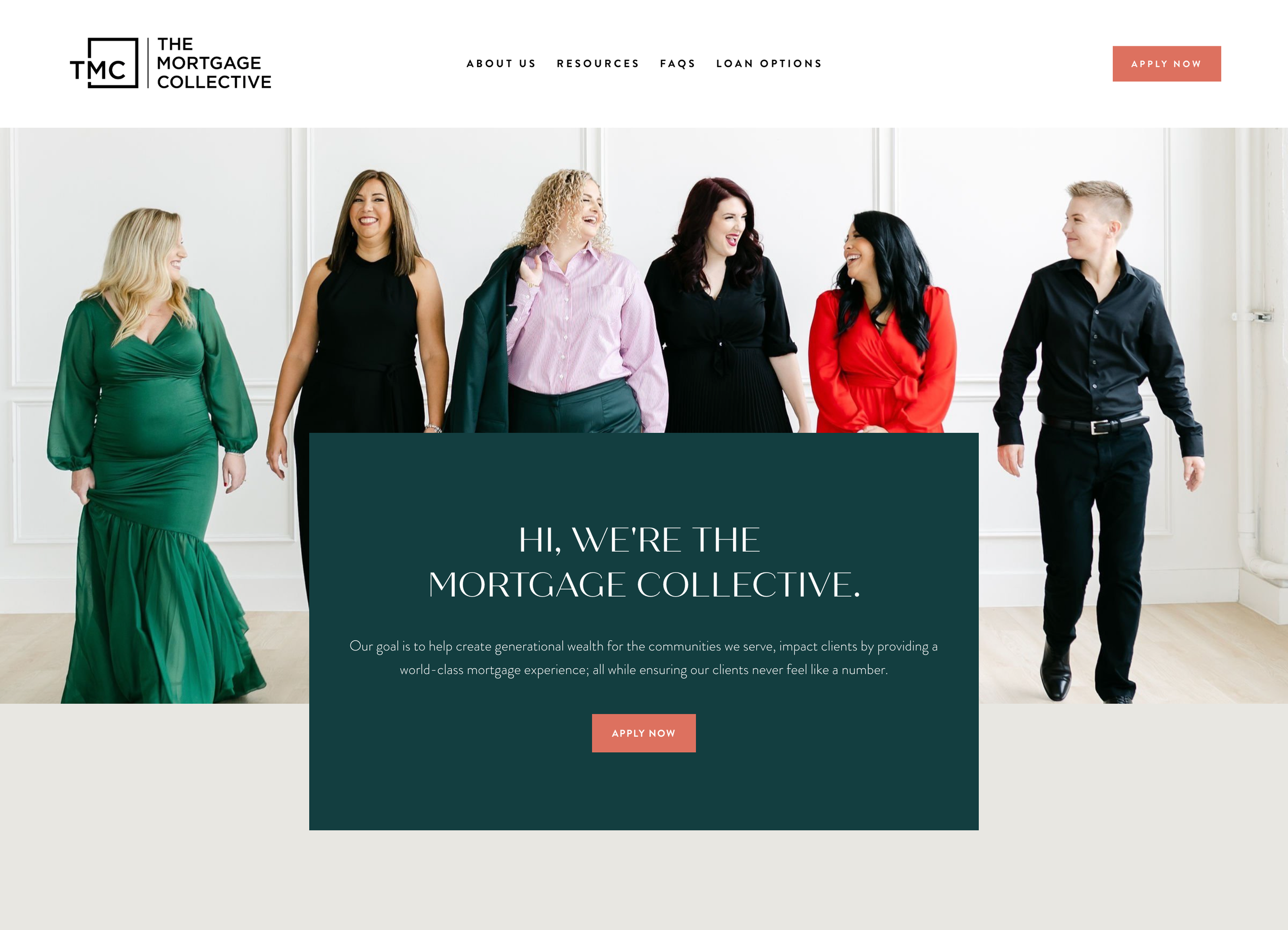The image features a prominent blue square logo in the top-left corner with the initials "TMC" representing "The Mortgage Collective." To the right of the logo, there are clear headings labeled "About Us," "Resources," "FAQs," and "Loan Options." Below these headings is a red rectangle button with white text that reads "Apply Now."

In the main section of the image, six individuals are lined up from left to right in front of a neutral background, providing a visual representation of the Mortgage Collective team. Starting from the left:

1. A woman wearing a green long-sleeve dress.
2. A woman in a sleeveless black dress.
3. A woman dressed in a green suit over a pink long-sleeve shirt, casually holding her suit coat over her shoulder.
4. Another woman in a mid-length sleeve black dress.
5. A woman in a red long-sleeve dress.
6. A man dressed in black pants with a black long-sleeve shirt.

The caption along the bottom of the image says, "Hi, we're the Mortgage Collective," written in white text on a bluish-green rectangle, accompanied by another "Apply Now" button.